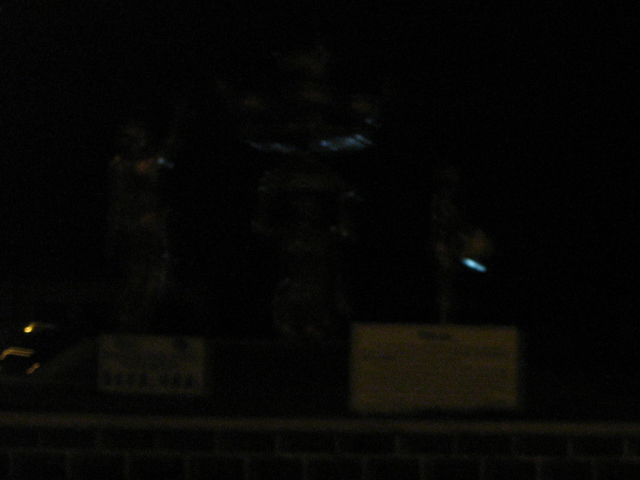The image is a photograph taken at night, resulting in a very dark scene with minimal illumination. The background is pitch black, suggesting it was taken either outside under a night sky or in a room devoid of light sources. In the center upper part of the image, there appears to be a glistening light, almost reminiscent of the night sky. The focal points are three statues, which are slightly illuminated and arranged from left to right across the image. 

On the left stands a statue, possibly holding a sword-like object, with a small yellowish illuminated sign beneath it, but the text is unreadable. This object is dark, with vague outlines hinting at a human figure. In the middle, another statue, potentially of a knight due to its silver-toned armor, faces directly towards the viewer. Beneath it, a sign with a white background and black text may indicate details about the statue, but the words aren't legible. 

On the center right, the third statue faces towards the right side of the image. This statue too has a sign underneath it, similar to the one in the middle, but it's not illuminating anything around it. The statues and signs are placed on a solid surface that might be a platform, which appears to be set upon a red brick wall spanning from the left to the right side of the image.